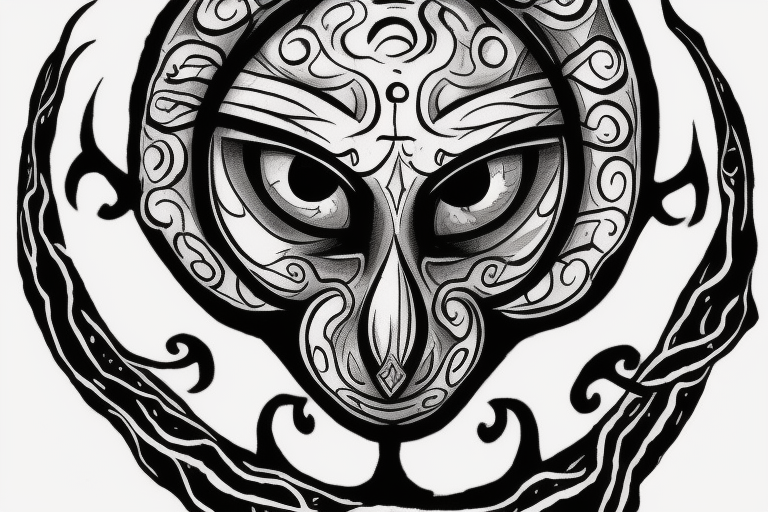This black-and-white tattoo design features a central face that resembles a mystical or tribal creature with almond-shaped eyes and a diamond-shaped nose. The face, which might evoke images of a stylized skull or a spirit of animal-like or ape-like appearance, has intricate, swirling patterns and curvy lines encircling it. These elements lend the design a dynamic, tribal border style. Beneath the face, there's a crescent moon motif, accompanied by additional crescent shapes and swirls, adding depth and complexity to the artwork. Made entirely in black, white, and shades of gray, the hand-painted drawing exudes an enigmatic, otherworldly aura and could be fixed to fabric as part of its ornamental appeal.